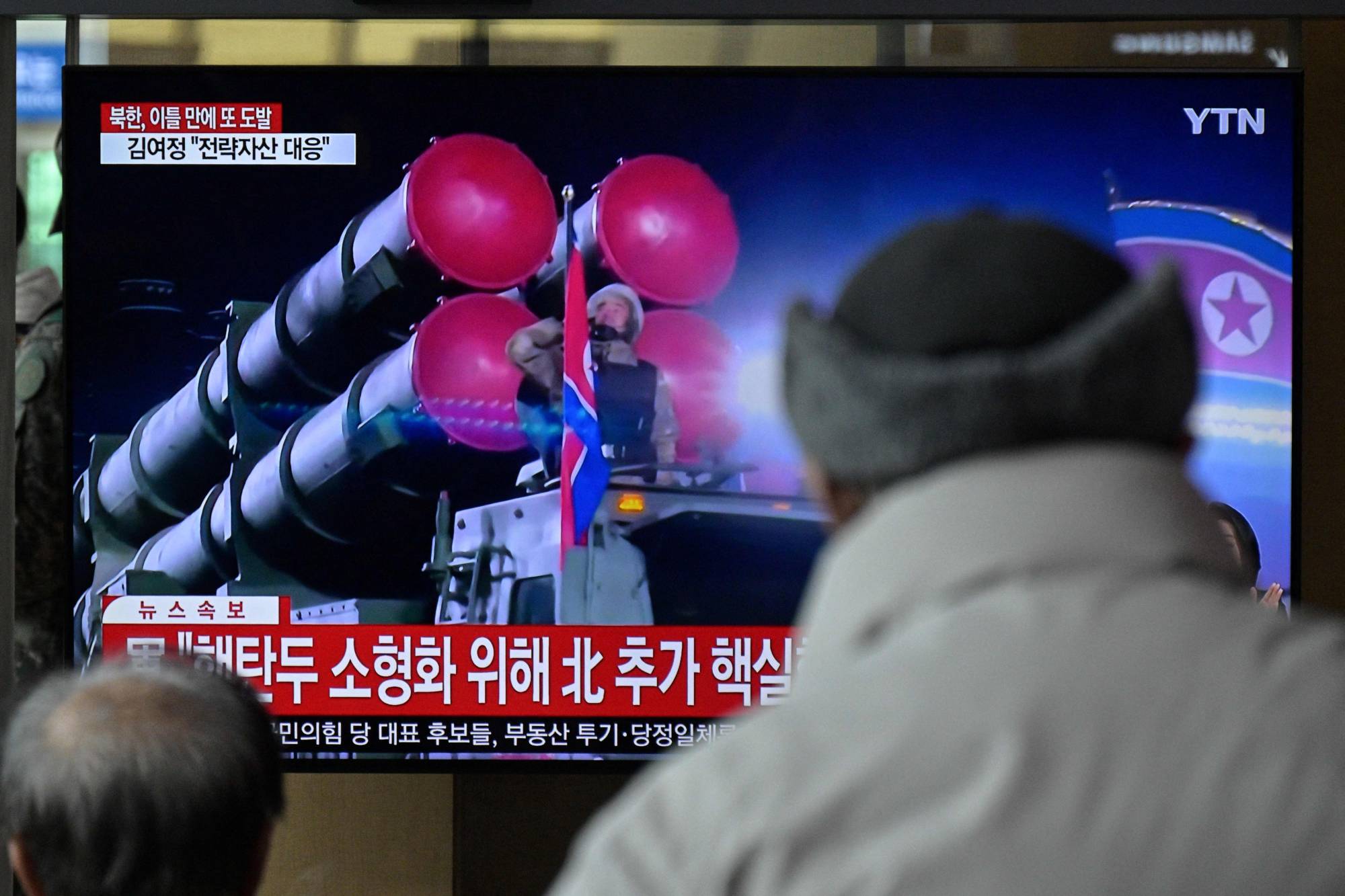The image depicts a large screen TV broadcasting a news segment, characterized by red and white Korean text, with a thinner line of white text on a black background underneath. The screen shows a soldier, who is in military uniform and saluting, on top of a massive truck carrying large, long missiles capped with red circles behind him. A partially visible North Korean flag with red, white, and blue hues and a star in the center is situated on the right side of the screen, along with the network identifier "YTN." In the foreground, the back of two individuals' heads can be seen. The individual on the left is shorter, balding, with dark brown and gray hair, while the one on the right is taller, wearing a gray hat and a khaki or off-white coat. They are positioned facing the screen, which also has flashes of windows barely discernible in the background, as they intently watch the broadcast.